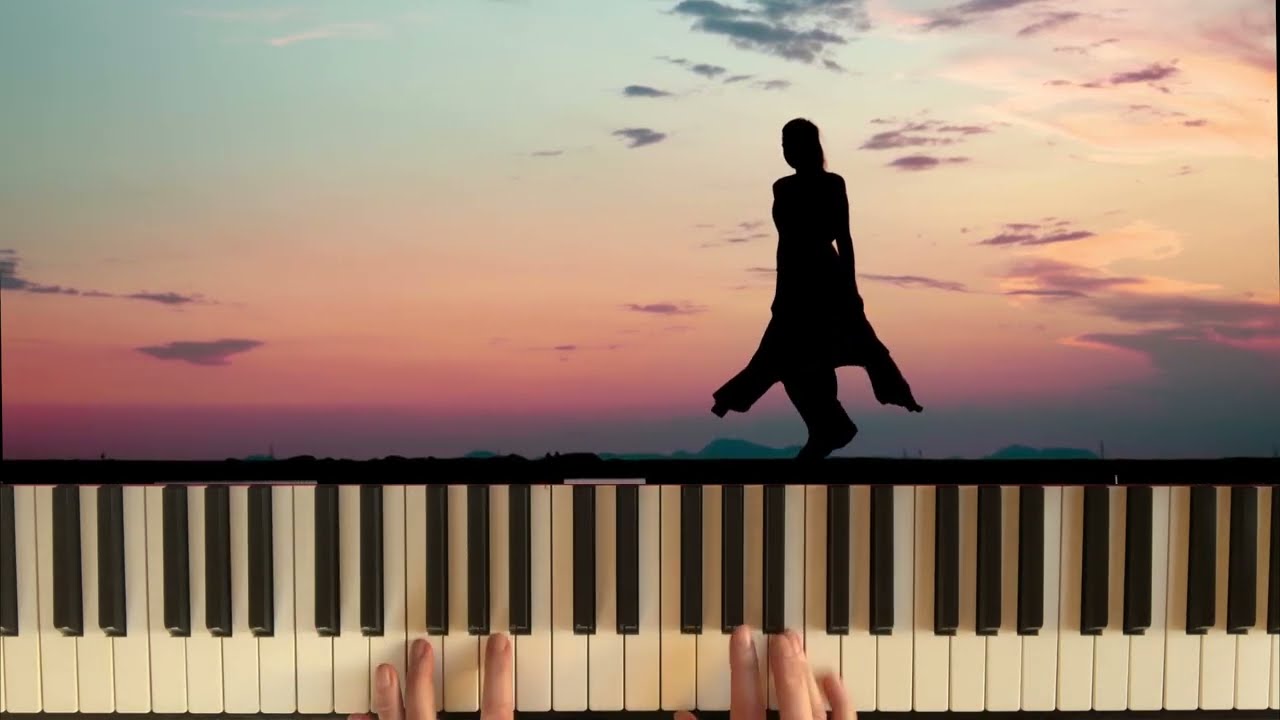The image is a photomontage consisting of two distinct sections. The bottom third showcases a piano from an overhead perspective, with visible black and white keys. Two hands are poised to play, with the left hand showing three fingers and the right hand displaying five fingers with the thumb partly visible. The top two-thirds depict a silhouette of a woman who seems to be either walking or dancing on a bridge or pier. She has long hair and appears to have a jacket or sweatshirt tied around her waist with loose fabric flapping on both sides. The sky behind her suggests a sunset or sunrise, transitioning from a light turquoise blue at the top to shades of peach, magenta pink, and purple, with some dark clouds. In the distant background, faint mountain lines are discernible. The woman’s direction seems to be aligned towards the piano player below her, integrating both the musical and scenic elements of the piece.